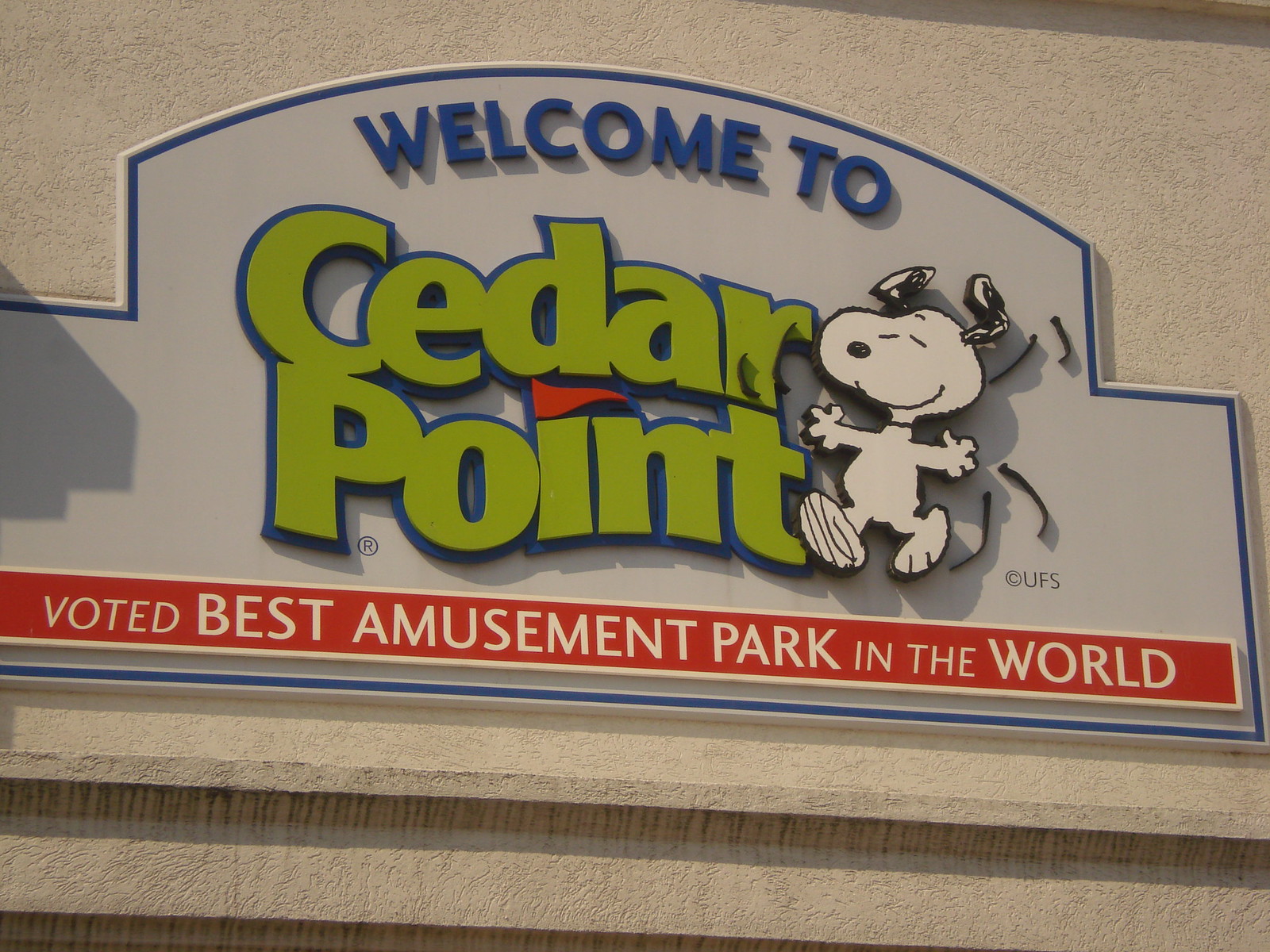The image is a horizontal rectangular photograph of a sign mounted on a white, concrete wall. The sign has a light blue background and is outlined by a darker blue border. At the top, the sign features an arching raised section that reads "WELCOME TO" in bold, blue capital letters. Beneath this, in green letters with a blue outline, it says "Cedar Point," with the dot over the "I" replaced by a small red flag. To the right of "Cedar Point," there is an illustration of Snoopy doing his happy dance, surrounded by small black motion lines. Lower on the sign, a long red rectangle in the bottom third states, "VOTED BEST AMUSEMENT PARK IN THE WORLD" in white font.